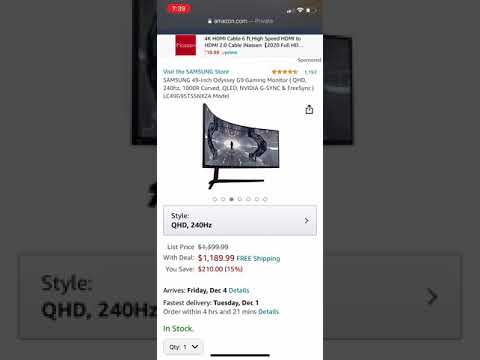This screenshot from Amazon.com showcases a product page for the Samsung Store. The featured item is a 49-inch Odyssey gaming monitor, known for its immersive curved QLED display. The monitor's extra-wide screen enhances the gaming experience by offering a more realistic and encompassing view. 

Listed specifications include QHD resolution and a 240Hz refresh rate, ideal for high-performance gaming. The current price after a 15% discount is $1,189.99, down from the original $1,399.99, offering a savings of $210. Free shipping is available, with an estimated delivery date of Friday, December 4th. For faster delivery, the monitor can arrive by Tuesday, December 1st, if ordered within the next 4 hours and 21 minutes. The item is in stock, as indicated by the green text, and the selected quantity is one. Additional details can be accessed by clicking next to the listed options.